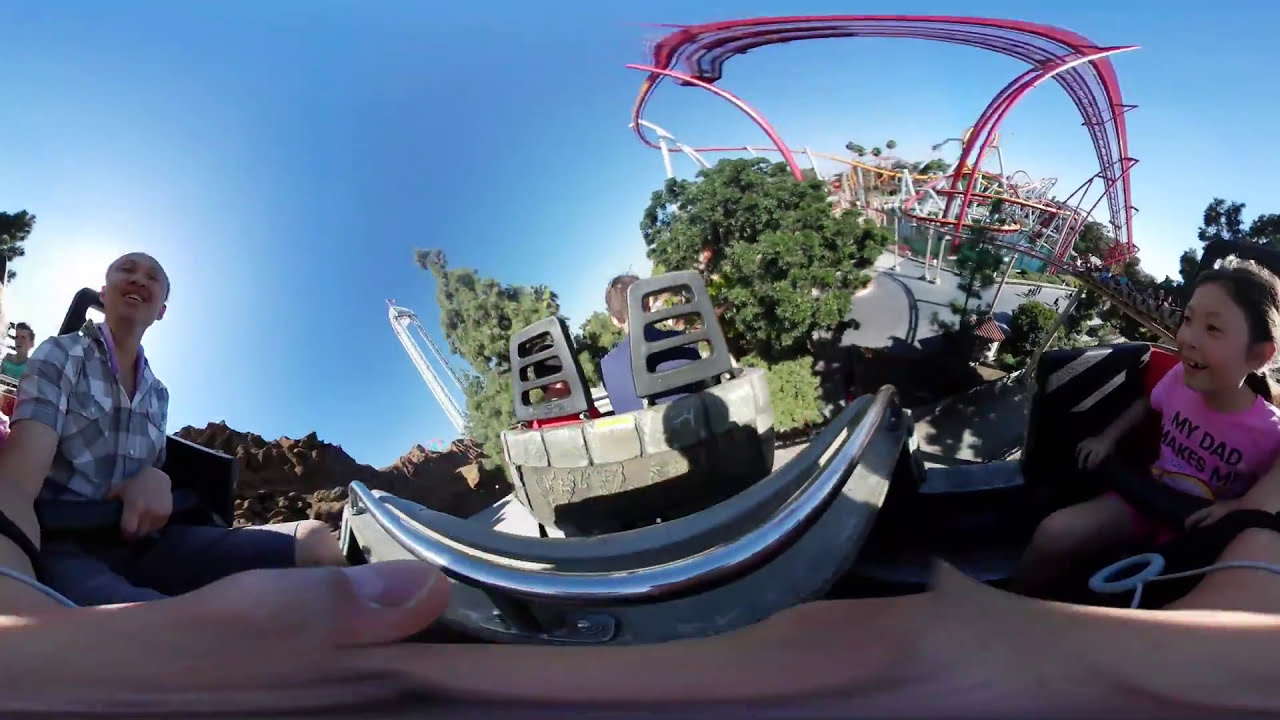In this captivating fisheye-style photograph, taken at an amusement park, we see a joyful scene on an outdoor roller coaster. Central to the image is a smiling young girl on the right, strapped securely into her seat and wearing a pink t-shirt emblazoned with the words "My Dad." Beside her sits an equally delighted man in a black, gray, and white checkered shirt who is capturing the moment with his camera. His arm, greatly distorted due to the lens, stretches towards the front of the frame, creating an unusual and striking effect. 

Behind them, other passengers can be seen seated, enjoying the thrilling ride. The roller coaster's vibrant red structure weaves through the image, contrasting with the vivid blue, clear sky above. Surrounding the ride, lush green trees add a natural backdrop, and in the far distance, hints of a tall white building and rolling hills add depth to this bustling amusement park scene.